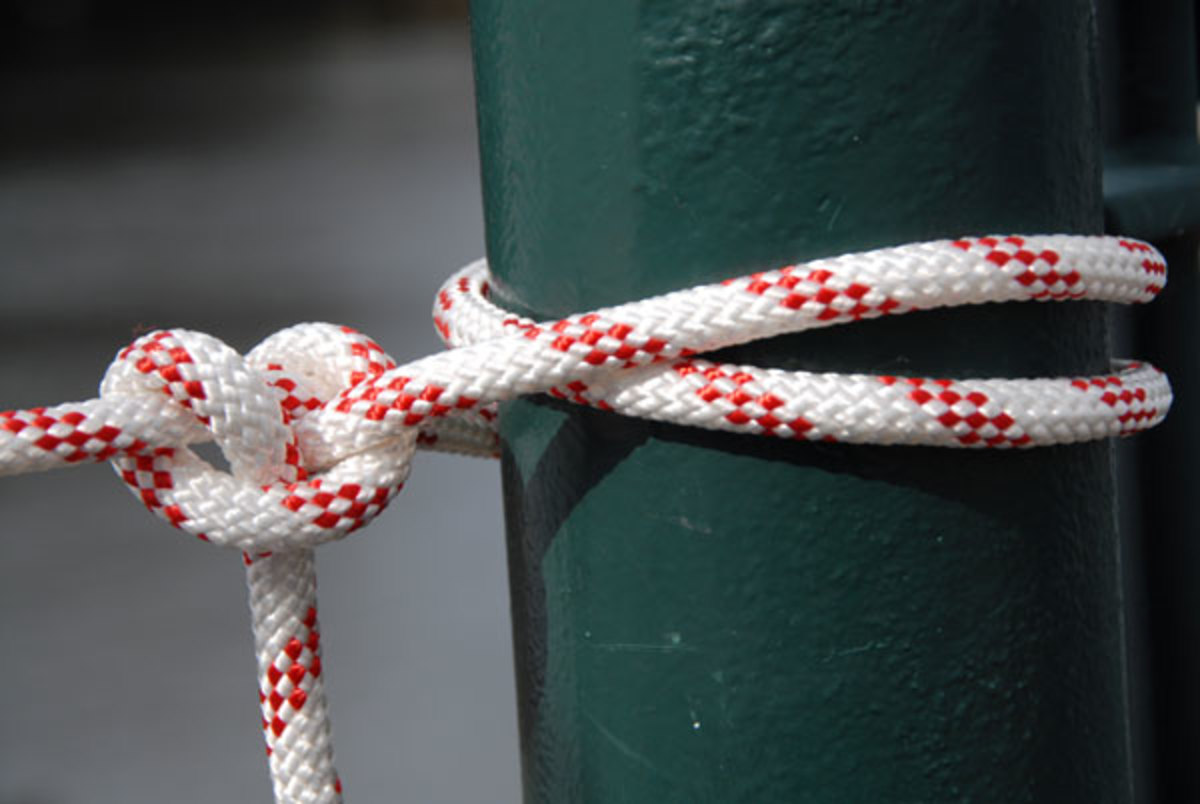The image depicts a detailed close-up of a nearly new red and white braided rope, expertly tied around a cylindrical, dark green painted pole, likely made of metal or possibly concrete. The rope, not particularly thick or thin, is wrapped twice around the pole and secured with a figure-eight knot, with one loose end trailing downwards. The pole, consistently dark green and possibly freshly painted, has some textural details but remains mostly smooth. The background is blurred, resembling a smooth, watery surface with various shades of gray and black, creating a slightly darker gradient towards the top left. The overall setup, with the green pole and contrasting red and white rope, stands out subtly against the indistinct backdrop.